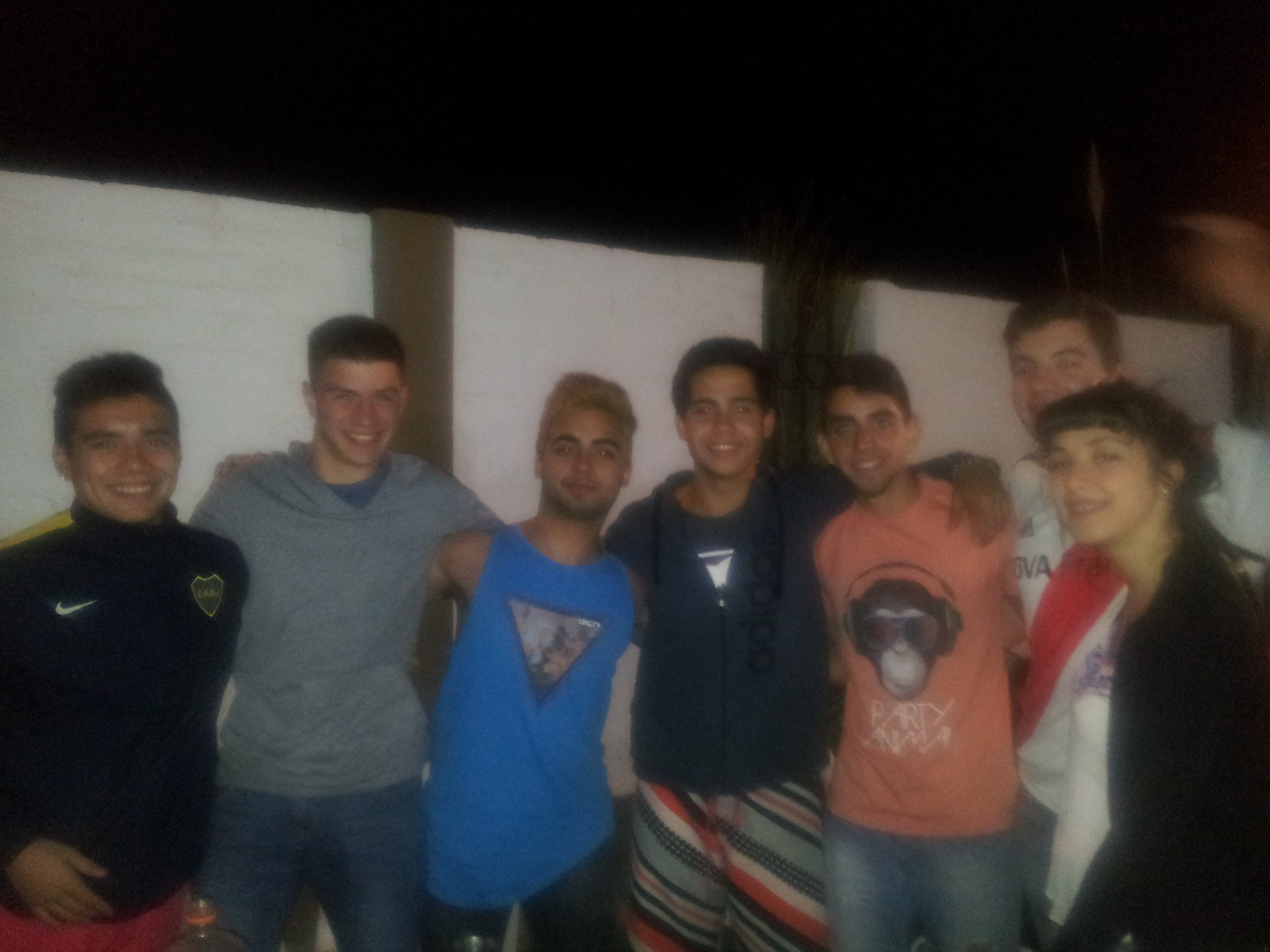This nighttime photograph captures a lively group of friends standing outside in front of a white wall, arms around each other and smiling brightly at the camera. There are eight people in the photo, consisting of seven males and one female. The female, positioned on the far right, is dressed in a black long-sleeve shirt, and she has dark hair. Her body is turned slightly to the side, giving us a side view of her figure and a full view of her smiling face.

To her left are the seven males, each distinguishable by their unique outfits and hairstyles. Starting from the right, closest to the girl, is a guy with short brown hair, wearing a white shirt featuring a red streak down the center, and he's smiling. Next to him stands a guy in an orange shirt adorned with a graphic of a monkey wearing glasses and headphones, paired with blue shorts. Following him is a male dressed in a black jacket and pants with swirling red, white, and blue stripes.

Positioned in the middle of the group is a guy in a blue tank top with blondish dyed hair and another with a gray hoodie and jeans. The next person, also in the center, wears a dark blue jacket—possibly a Nike jacket— and has short hair. All of them showcase a wide array of styles, adding to the picture's vibrant atmosphere.

The sky is visible above the white wall, hinting at the calmness of night, and a small cloud can be spotted in the top right corner. Every person in the photograph is looking at the camera, united by their joyful expressions and the camaraderie evident in their body language.